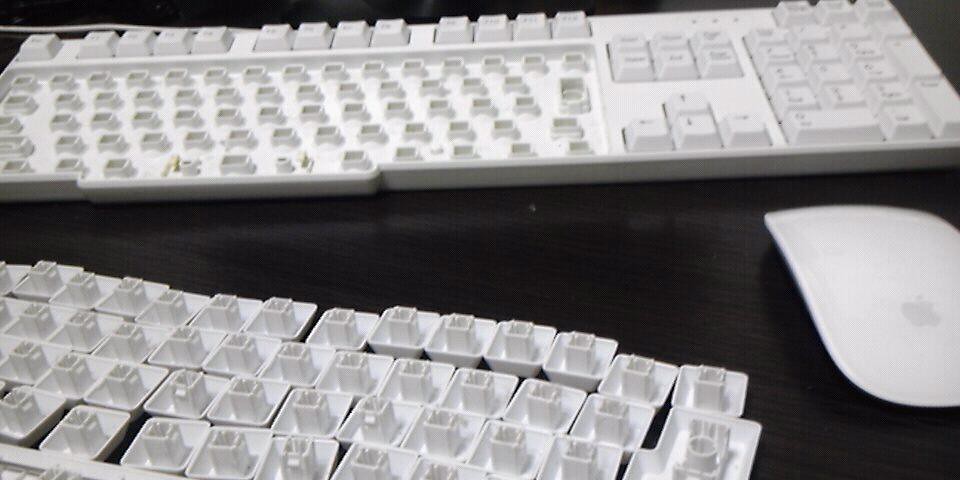The image depicts a detailed scene of a keyboard on a sleek, shiny black wooden desk. The white keyboard takes up the upper half of the image, with a thin silver wire visible in the top left corner. Most of the keys from the main typing area have been removed, revealing the empty sockets where the keys would normally be. However, the F-row, arrow keys, and number pad remain intact. In front of the keyboard, aligned in an organized fashion, are the removed keys, all turned upside down to expose the inserter pieces. To the bottom right of the image, there is a white Apple mouse with a faint grey Apple logo. The photograph captures the meticulous arrangement on the glossy black surface, suggesting a process of keyboard repair or cleaning.